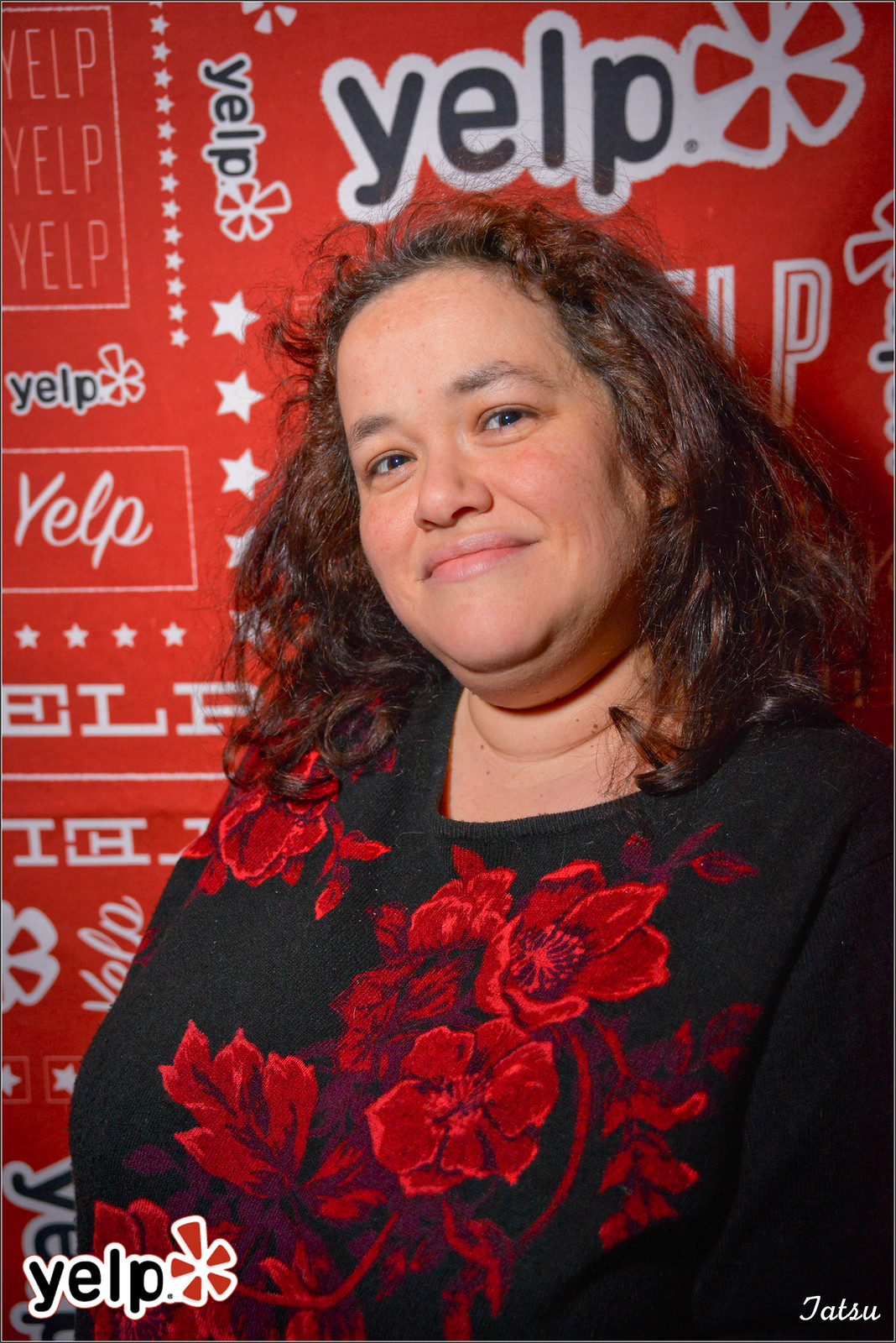The image is a vertical close-up photograph of a woman with an auburn, wavy, and slightly unkempt shoulder-length hair. She has a lighter brown skin tone and is likely in her late twenties to early thirties. The woman is wearing a black top with large red flowers as the design, which might be a dress or sweater. Her head is tilted to her right, and she has a partial, closed-mouth smile. The background is entirely covered by a banner with a repeating Yelp logo in various fonts and sizes, incorporating both black and red text along with white stars and flower designs. The primary Yelp logo appears in the bottom left corner, and the name "Tatsu" spelled T-A-T-S-U, is visible in the lower right corner. The predominant colors in the image are black, white, and red, and no other people or animals are present.